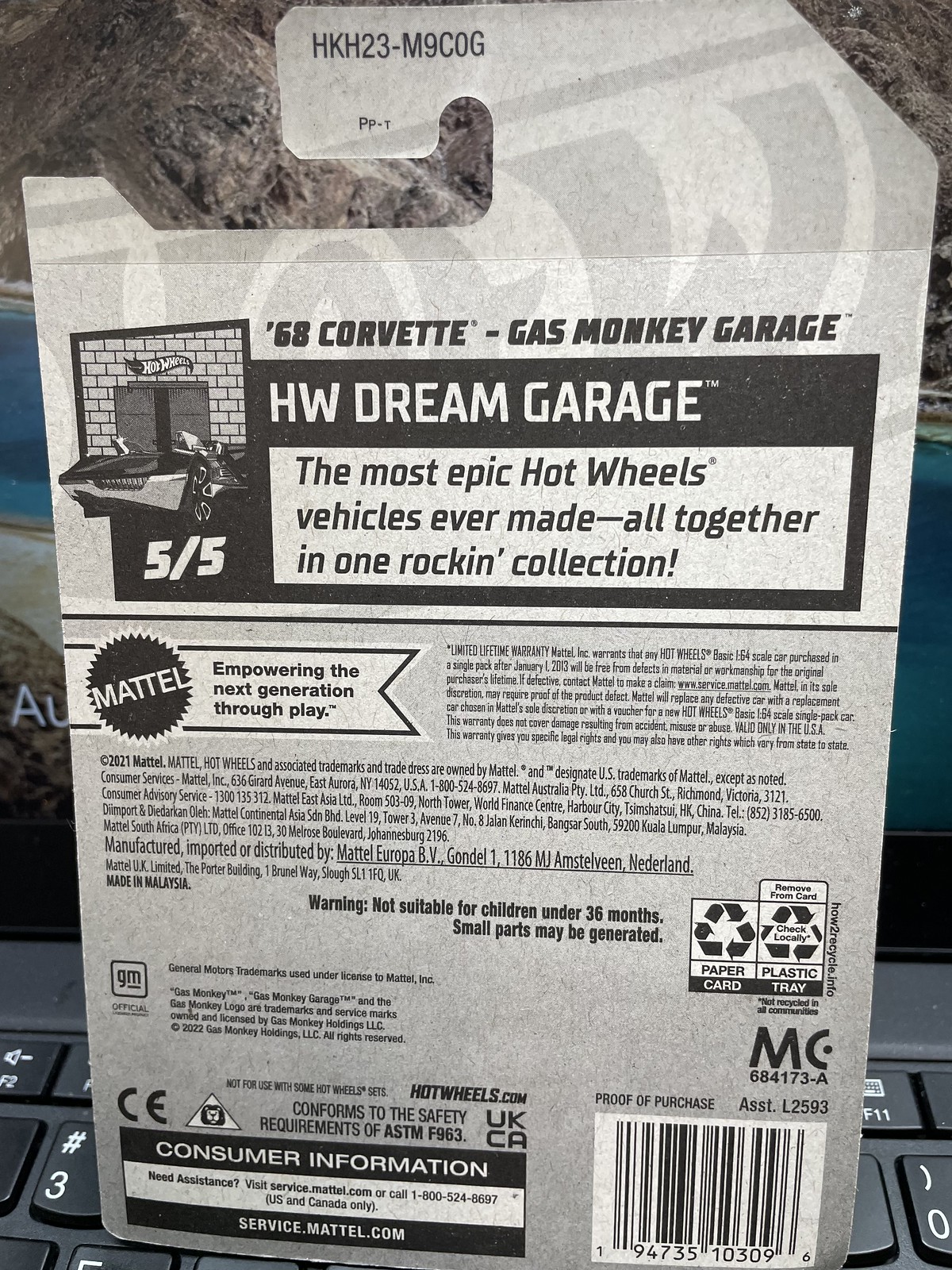The image displays the back packaging of a Hot Wheels toy car, specifically a '68 Corvette from the Gas Monkey Garage. The packaging is placed on the keyboard of an open laptop, which has a black keyboard with the placard situated in front of the number keys. At the top of the cardboard packaging is a classic hang tab typically used for displaying items in stores. Prominent text at the top reads "68 Corvette Gas Monkey Garage," followed by "HW Dream Garage" in large lettering. Below, within a white rectangle, it states, "The most epic Hot Wheels vehicles ever made all together in one rocking collection." There's a small illustration of the Hot Wheels car on the left side. Additional details include the Mattel logo and various informational texts such as limited lifetime warranty, Mattel's address, and recyclable symbols. A barcode is clearly visible in the bottom right corner, while consumer information is listed on the bottom left. The packaging is primarily gray and resembles typical Hot Wheels packaging material.